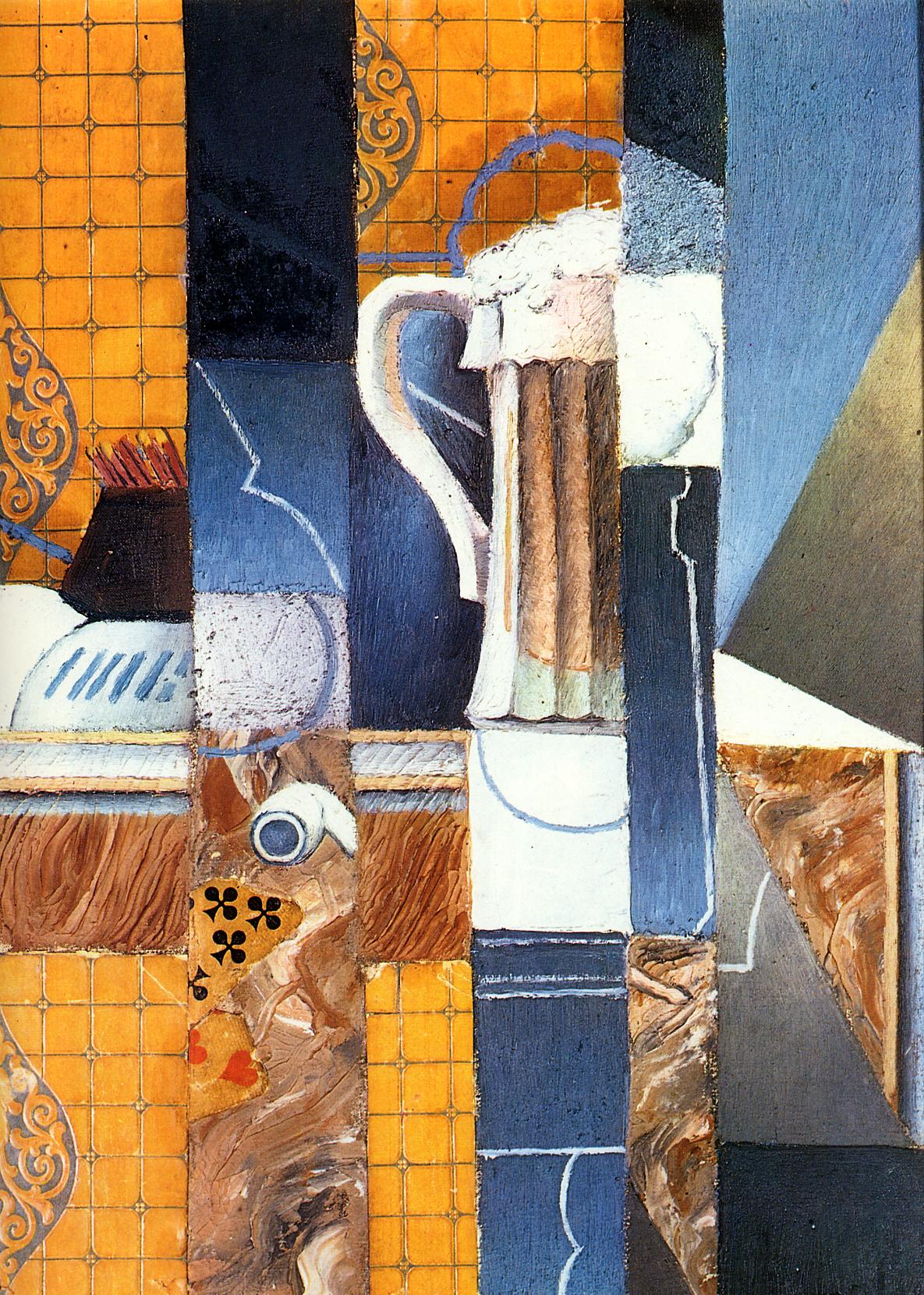The painting in the image is a detailed and colorful abstract collage composed of five vertical sections, each filled with various shapes, patterns, and colors. Set against a predominantly yellow background featuring square-like tiles, the painting is divided into intricate subsections. The first vertical segment features a dark upper section with red accents, transitioning to bluish and brown hues below. The second segment showcases alternating light and dark blues with a white, crooked line and a blue half-moon. This area also contains a multicolored portion with brown tones, black designs, red hearts, and white headphone-like shapes. 

In the third segment, scattered dark blue sections intermingle with yellow squares and designs, leading to an image of a half-visible beer mug. The fourth section, narrower than the others, alternates between dark blue, light blue, white, and brown areas with intricate patterns. Lastly, the fifth section displays a majority blue field, interrupted by green and white triangles, as well as brown and-gray diagonal divisions ending in a dark blue rectangle.

Throughout the collage, there are recurring shapes like cups, a half-cut pizza, and overlapping triangles, primarily in blue, grey, and brown hues. The overall composition melds floral designs with geometric forms in a symphony of colors—ranging from vibrant yellows and oranges to subdued blues and browns—creating a complex and engaging visual narrative.